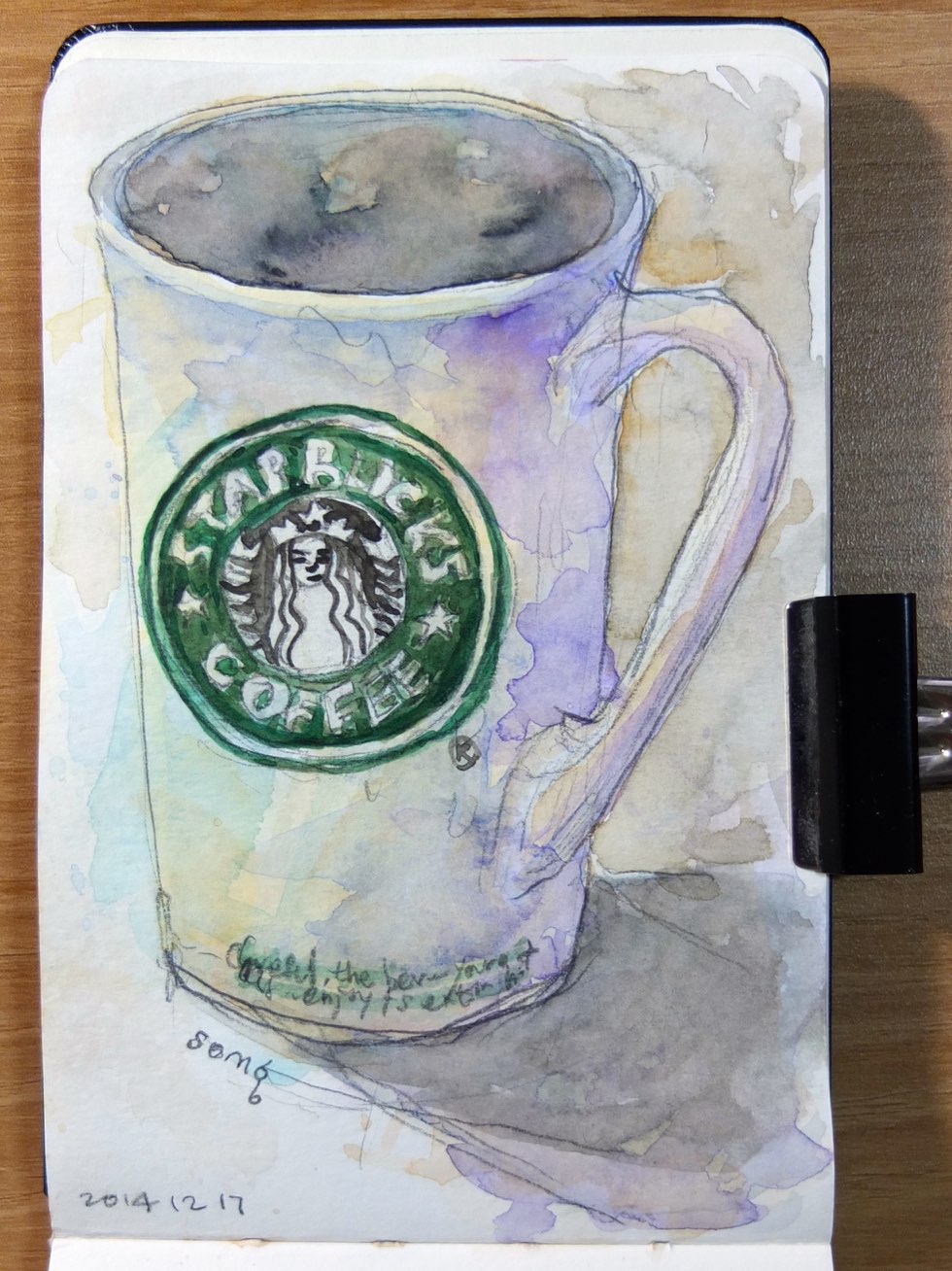A captivating artwork combining pencil sketch and watercolor portrays a meticulously rendered mug and beaker featuring the iconic Starbucks coffee logo. This exquisite piece showcases the artist's skill through the delicate freehand pencil work that outlines a tall mug with a smooth handle. The Starbucks logo, with its crowned female figure, is reinterpreted with intricate detail, anchoring the center of the composition. The background is a spirited array of splotches and swirls, reminiscent of an impressionistic style, adding depth and a dynamic sense of movement. At the bottom of the piece, the date 2014, 12, 17 is inscribed, possibly indicating the artwork's creation date. Additionally, the image appears clipped to the edge of a surface, likely a pad or a cell phone, against a backdrop showing wood grain texture, enhancing the overall organic and tactile quality of the presentation.